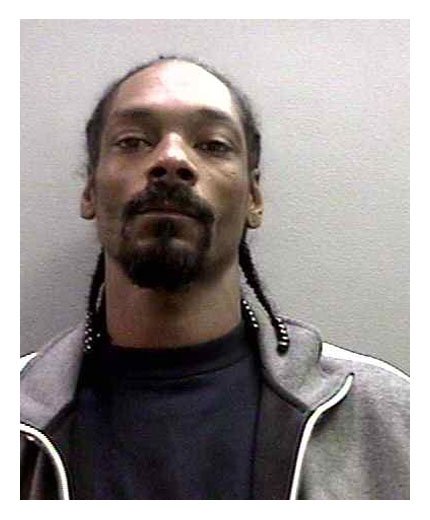The image is a casual portrait of the rapper Snoop Dogg, also known as Calvin Broadus, taken from a slightly upward angle. Snoop is leaning against a grey wall and looking down towards the camera, giving a slightly menacing yet typical Snoop expression. His hairstyle features three to four black braids, adorned with black beads at the tips, hanging down to his shoulders, while the rest of his hair is short. He sports his usual Van Dyke-style mustache and goatee. Clothing-wise, Snoop is dressed in a light grey jacket with a black lining, left open to reveal a dark navy blue workout t-shirt underneath. The picture is closely framed, capturing him from the mid-chest up, with no other people or context visible in the background.